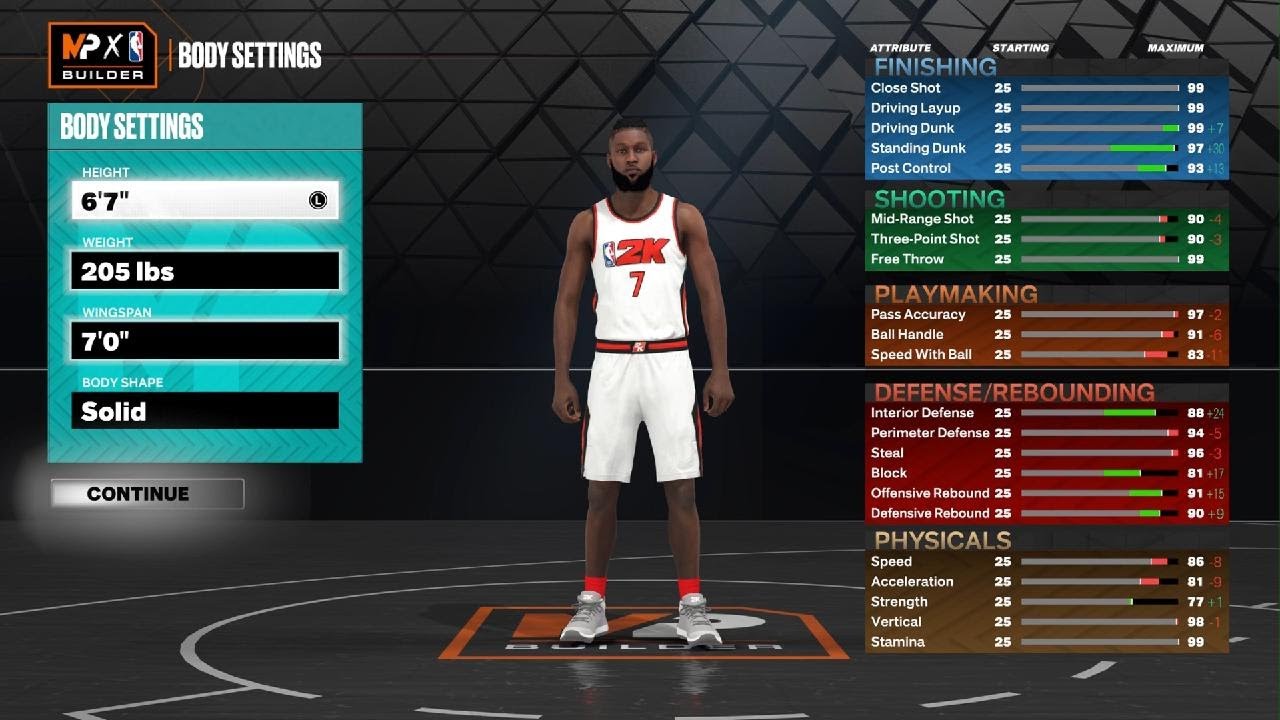In this screenshot from an NBA video game, the screen header reads "MPX Builder" at the top. The primary focus is an African-American player donning a jersey, showcased in the center of the screen. The player features black hair, a faint beard, a slight goatee, and a barely noticeable mustache. 

To the left, a panel titled "Body Settings" is set against a teal background adorned with raised lines. In white text, this panel lists customizable attributes including height, set at 6'7", weight at 205 lbs, wingspan at 7'0", and body shape labeled as "Solid." A "Continue" button is also visible below these settings.

On the right side of the screen is another panel labeled with the attributes: "Starting" and "Maximum." Categories listed here include "Finishing," "Shooting," "Playmaking," "Defense/Rebounding," and "Physicals," each accompanied by numerical values. The initial values in the first row are all set to 25. The first box at the top is blue, "Shooting" is green, "Playmaking" and "Defense/Rebounding" are red, and "Physicals" are green, providing a color-coded system for easy reference.